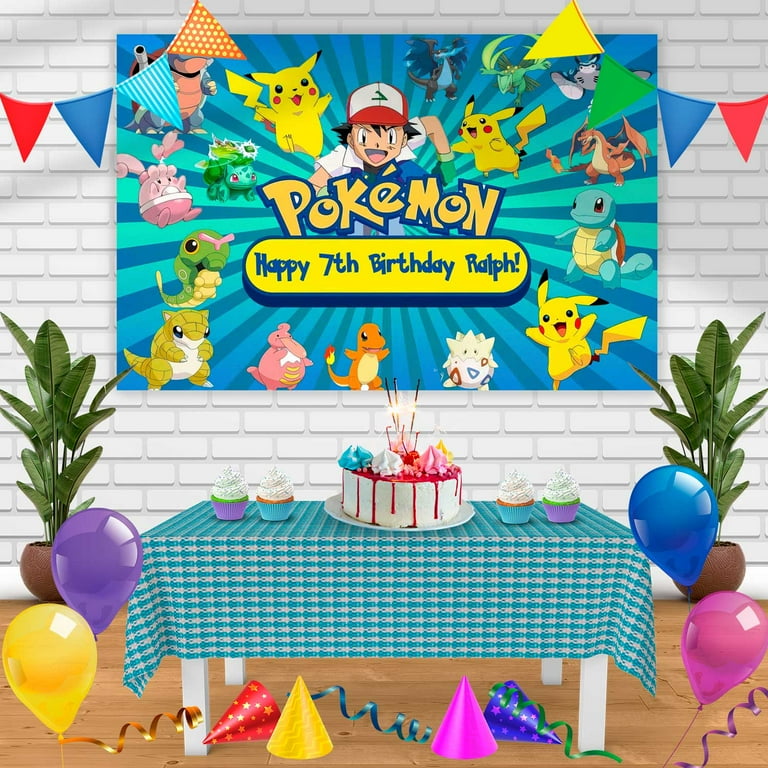The image is a vibrant cartoon scene depicting a child's birthday party setup. Central to the scene is a long table with white legs, draped in a turquoise and white checkered tablecloth. The table features a variety of confections including a centerpiece—a large white cake adorned with red icing, candles, and colorful floral decorations. Flanking the cake are six cupcakes, with two on either end and four clustered in the middle. Behind the table, against a white brick wall, hangs a large celebratory poster exclaiming, "Pokemon, Happy 7th Birthday Ralph," surrounded by Pokémon characters and blue, radiating stripes.

On either side of the poster are decorative flags. Below the table, on the floor, are four party hats in red, yellow, purple, and blue, situated between sets of balloons in pink, blue, and yellow hues. Additionally, on both the left and right, near the balloons, are green potted plants—one in a vase with a fern-like plant growing and the other labeled as planters. This festive and colorful illustration perfectly encapsulates the excitement and joy of a Pokémon-themed birthday celebration.